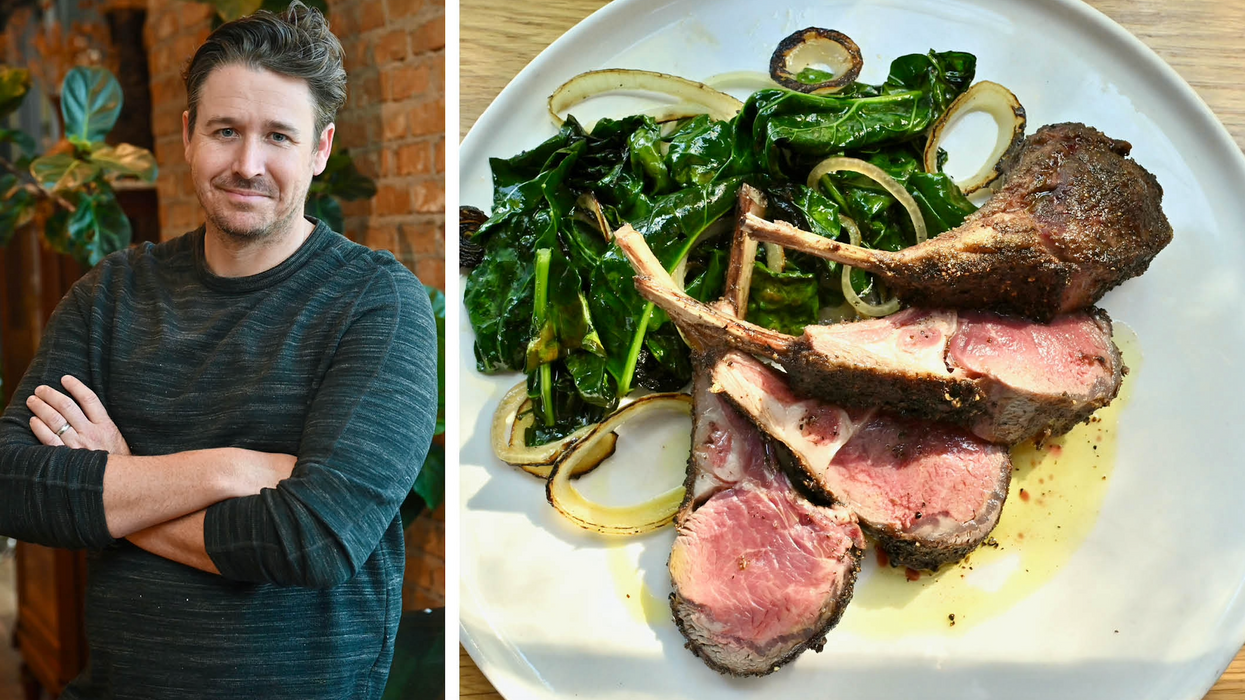This image features two side-by-side photographs that accompanied an article in a local Houston, Texas newspaper about the restaurant Ostia. The left photograph showcases Travis McShane, the owner and chef of Ostia. McShane, a Caucasian male in his late 30s to early 40s, stands confidently with his arms crossed in front of a brick wall. He is dressed in a dark green pullover sweater and sports a short haircut with a five o'clock shadow. His friendly demeanor is complemented by a pleasant smile.

The right photograph highlights one of McShane's culinary creations: a beautifully plated meal consisting of four thin lamb chops. The lamb chops, cooked to a perfect medium with a pink interior and a crusted exterior, are artfully arranged on a white plate with the bones elegantly fanned out. Surrounding the lamb chops is a bed of vibrant green sautéed spinach mixed with grilled onions, lightly drizzled with oil. This dish, known as a rack of lamb, showcases the refined culinary skills and attention to detail that characterize the dining experience at Ostia.